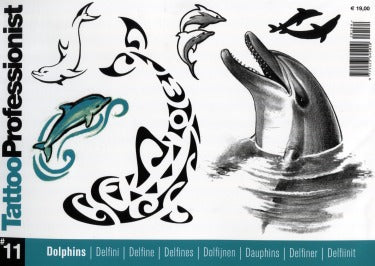The image depicts the cover of a tattoo design book aimed at professional tattoo artists. The background is a light grayish-white. Along the left side, text runs vertically, with "tattoo" in aqua and "professionalist" in black. Various dolphin illustrations populate the center of the cover. These include detailed drawings: a black pencil-shaded dolphin emerging from the water, a tribal tattoo-style dolphin, two dolphin silhouettes connecting, and an outlined dolphin with an aqua blue center and swirling waves. In the upper right corner, there is a black barcode. At the bottom, a horizontal strip features a black square with the number "11" in white text and an aqua square with "dolphins" in white text. The word “dolphins” also appears in multiple languages along the strip.